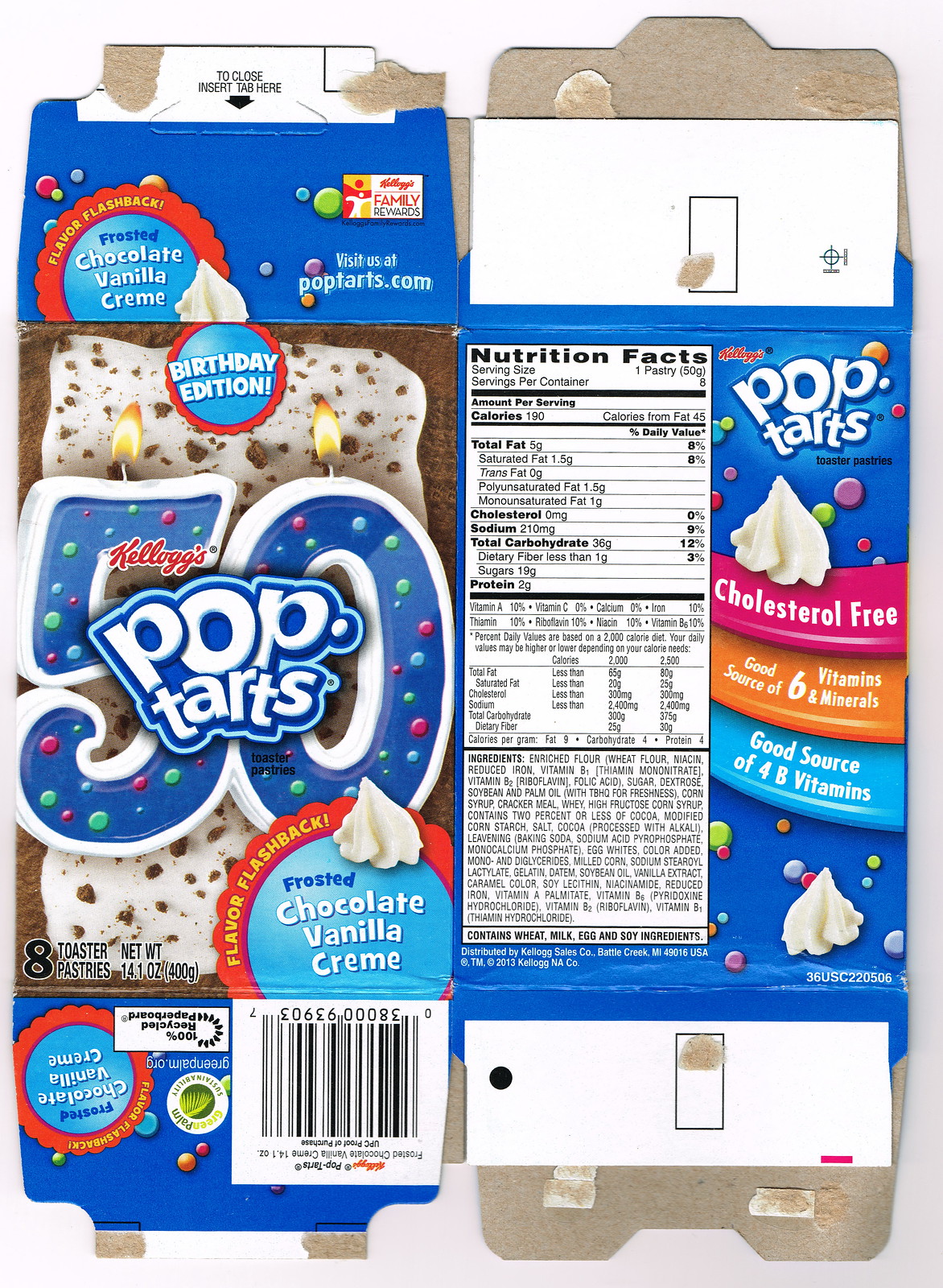This image features a smashed blue box of Kellogg's Pop-Tarts, specifically the Frosted Chocolate Vanilla Cream variety, celebrating the brand's 50th anniversary. The front of the box prominently displays the product along with several labels, including "Birthday Edition," "Cholesterol-Free," "Good Source of Six Vitamins and Minerals," and "Good Source of Four B Vitamins." Additionally, the barcode is visible at the bottom of the front side of the box. Due to the flattened nature of the box, the back is also visible, showing the nutritional facts.